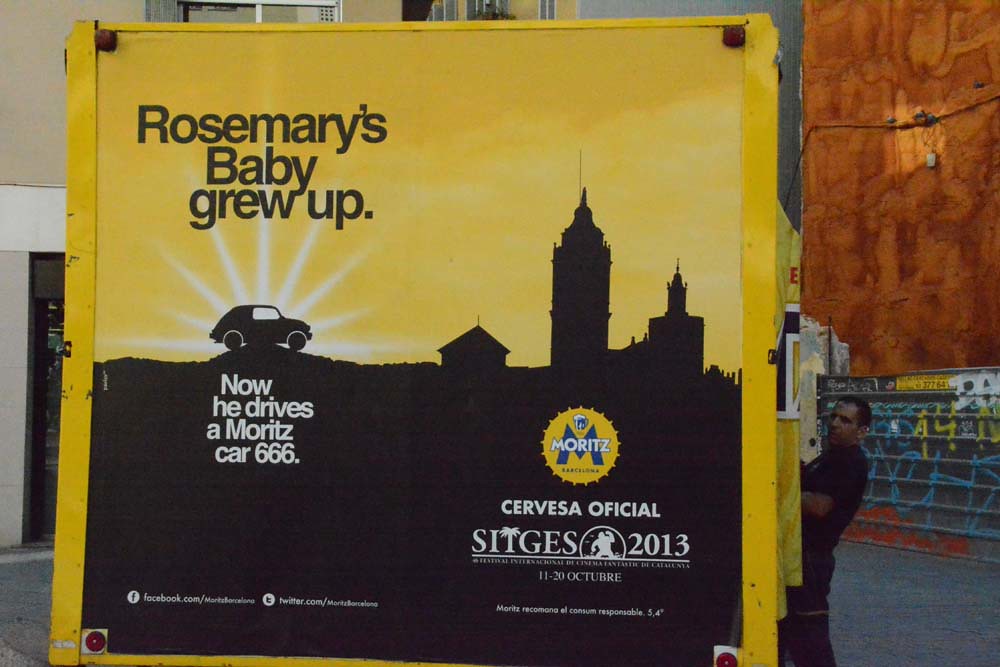In this outdoor photograph, the back of a mostly yellow truck features a detailed promotional ad. Dominating the ad is a graphic design silhouette of a small town with black buildings and a black car. Positioned over a radiant sunset background, black text announces, "Rosemary's Baby Grew Up." Just below the car, against a black background, white text reads, "Now he drives a Moritz Car 666." To the right of the car, a yellow stamp or logo depicting a black "M" and the text "Moritz" is visible. Beneath the logo, the ad states "Cerveza Oficial" in white writing with the year "2013" and an image of a man. A person stands nearby, enhancing the scene's depth and scale.